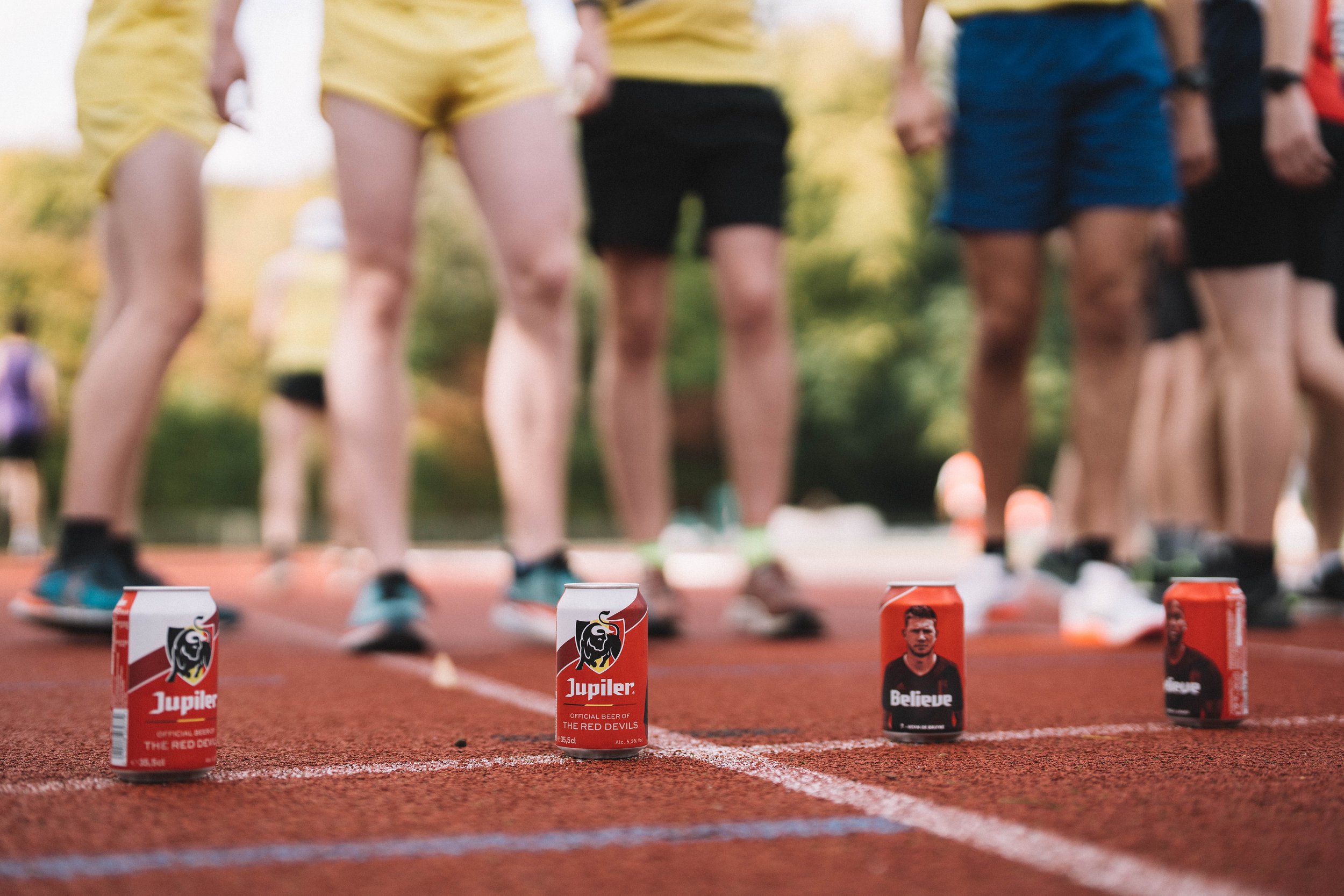This image is a landscape-oriented color photograph taken at ground level, capturing a red running track with several white and gray lines. Lined up across the track are four cans of beer, specifically the brand Jupiler, spelled J-U-P-I-L-E-R. The cans, which are the size of standard soda cans, feature a predominantly red design with a dark red and white swirl pattern. Each can has a shield logo with a black bull prominently displayed. The text at the bottom reads "The Red Devils," indicating it is the official beer of the Red Devils. 

The leftmost two cans show the brand logo prominently, while the two on the right include images of people – one depicting a white man and the other a black man – with the word "Believe" in white text beneath their images. In the blurred background, several runners, dressed in a variety of colored running shorts and shoes, wait to start a race. The runners' socks vary between dark and white, and beyond them, there are hints of trees and additional blurred figures. This composition focuses on the contrast and positioning of the beer cans against the dynamic yet out-of-focus backdrop of the track and runners.